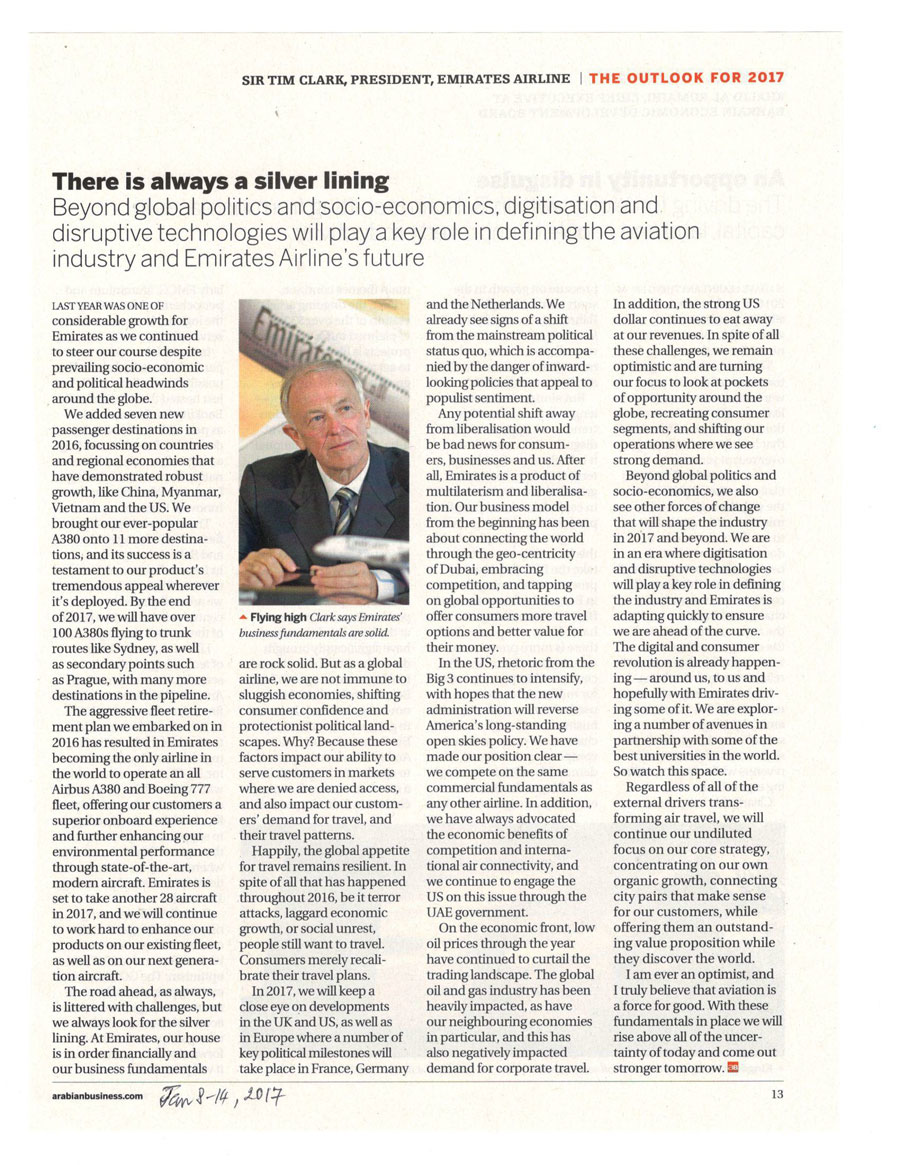This is a detailed caption of a photograph taken of a magazine page, possibly showing some discoloration due to the photography. The background of the page is cream-colored. At the top right corner of the page, the text reads, "Sir Tim Clark, President, Emirates Airline." Adjacent to this, in red font, is the title "The Outlook for 2017."

In the bottom right-hand corner is the page number "13." On the left side of the page, there's a tiny, unreadable website address. Handwritten on the page is the date "January 8 to 14, 2017."

The headline of the article on this page states, "There is Always a Silver Lining." Below this bold headline, there is a subheadline in regular font, which reads, "Beyond Global Politics and Socioeconomics, Digitization and Disruptive Technologies Will Play a Key Role in Defining the Aviation Industry and Emirates Airline's Future."

The article is composed of four columns of dense text. At the top of the second column from the left, there's a photograph of an older white man dressed in a suit. The background of this photograph features what appears to be a rolled-up newspaper with "Emirates" prominently displayed as the headline.